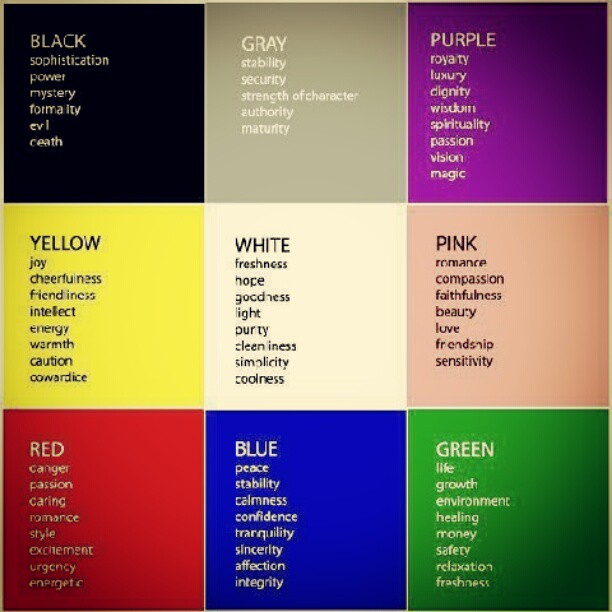The image features a square composed of nine smaller squares arranged in a 3x3 grid. Each smaller square is a different color, and each color is labeled in white text with descriptive adjectives associated with it. From the top-left to bottom-right, the colors and their corresponding adjectives are:

1. **Black:** Sophistication, power, mystery, formality, (blurry text).
2. **Gray:** Stability, security, strength of character, authority, maturity.
3. **Purple:** Royalty, luxury, dignity, wisdom, spirituality, passion, vision, magic.
4. **Yellow:** Joy, cheerfulness, friendliness, intellect, energy, warmth, caution, cowardice.
5. **White:** Freshness, hope, goodness, light, purity, cleanliness, simplicity, coolness.
6. **Pink:** Romance, compassion, faithfulness, beauty, love, friendship, sensitivity.
7. **Red:** Danger, passion, caring, romance, style, excitement, urgency, energetic.
8. **Blue:** Peace, stability, calmness, competence, tranquility, sincerity, affection, integrity.
9. **Green:** Life, growth, environment, healing, money, safety, relaxation, freshness.

Each word is vertically aligned beneath its corresponding color label, neatly depicting the various emotional and symbolic connotations associated with each color.